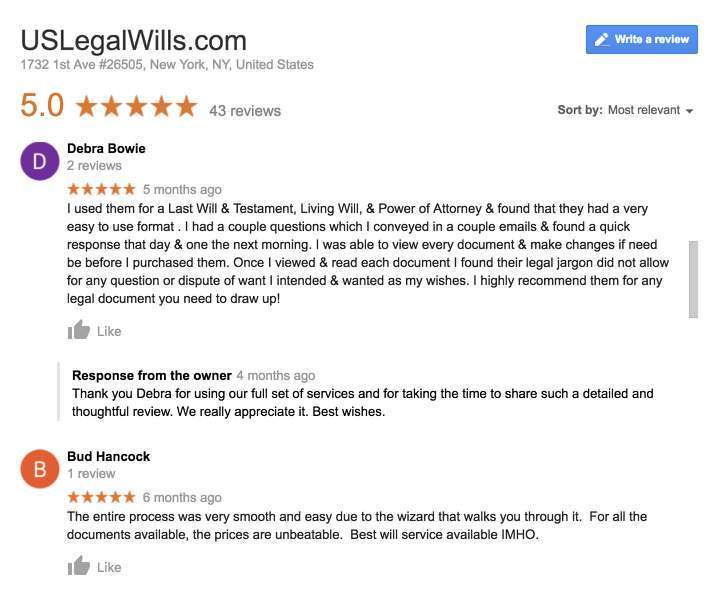**Detailed Descriptive Caption:**

The image displays a section of the website, uslegalwills.com, prominently showing its name in bold at the top left corner. Beneath the website name is the address: "1732 First Avenue, #26505, New York, New York, United States." This is part of a review section. The page exhibits a total of 43 reviews, highlighted by two prominent five-star reviews, with the 5.0 rating and accompanying stars in a vivid orange font. To the side, there's a blue "Write a Review" button featuring a white pencil icon and a squiggly line.

On the right side, beneath the "Write a Review" button, is a sorting option labeled "Sort by Most Relevant" in bold, accompanied by a drop-down triangle icon. The first review is from Deborah Bowie, marked by a white 'D' within a purple circle. Deborah praises the service, mentioning her use of it for a Last Will and Testament, living will, and power of attorney. She emphasizes the user-friendly format, quick email responses, and the ability to review and amend documents before purchase. She found the legal language clear and unambiguous, highly recommending the service for legal document preparation. Below her review is a thumbs-up icon, followed by a response from the owner, thanking Deborah for her detailed feedback.

The second review, from Bud Hancock, is indicated by a white 'B' within an orange circle. Bud gives a one-review, five-star rating, noting the smooth and easy process facilitated by the website's wizard tool, competitive pricing, and stating it's the best will service in his humble opinion. This review is also accompanied by a thumbs-up icon and a like button.